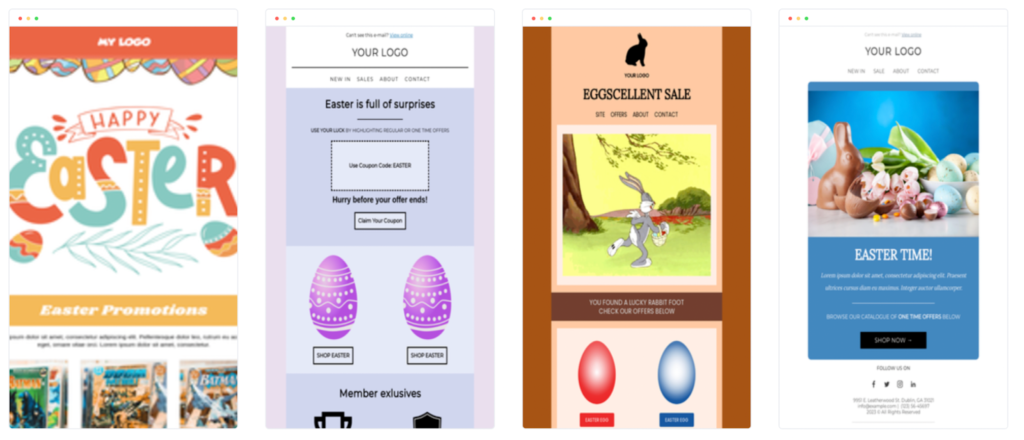The image showcases a vibrant Easter-themed page divided into four distinct sections, each highlighting festive elements and promotions.

1. The first section, titled "Happy Easter," prominently displays a logo and the phrase "Easter promotions." The color palette here features shades of red, tan, and light blue, creating a warm and inviting atmosphere.

2. The second section reads "Easter is full of surprises" and includes a different logo. It features two purple Easter eggs adorned with intricate white designs. There are captions beneath each egg, though the text is quite small and difficult to read. The background of this section is primarily light purple, complemented by accents of light blue and white.

3. The third section announces an "egg-cellent sale" accompanied by a black silhouette of a bunny rabbit. This playful section also includes an image of Bugs Bunny strolling through a forest scene, set just above a pair of brightly colored eggs—one red and one blue.

4. The final section, again marked with a logo, includes some small, hard-to-read letterings. This part features a delightful pairing of a chocolate bunny and a broken chocolate egg. The caption "Easter time" adds to the festive mood, all set against a calming blue background.

Each section is meticulously designed to capture the joyful and surprise-filled essence of Easter.